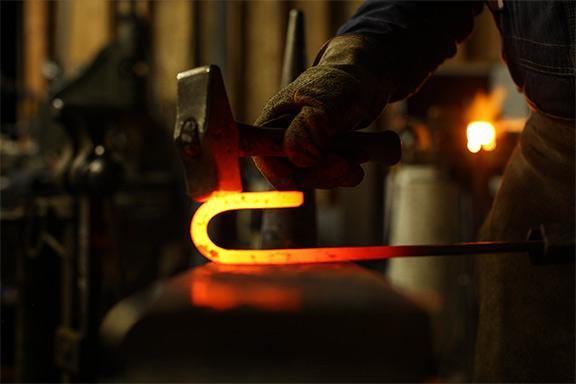The photograph showcases a skilled metalworker engaged in shaping a red-hot piece of metal, glowing brightly in shades of yellow and orange. He is intently focused on his task, wielding a heavy metal hammer in his right hand and wearing heavy-duty gloves, indicative of the extreme temperatures involved. The metal, formed into a candy cane-like shape, rests on a small anvil as he strikes it precisely at the curve. Behind him, a bright furnace illuminates the background, emphasizing the heat and intensity of his work environment. The overall scene is enriched with warm colors such as yellow, orange, red, and accents of black, gray, and brown, all set against a backdrop softly blurred to maintain focus on the craftsman and his meticulous process.